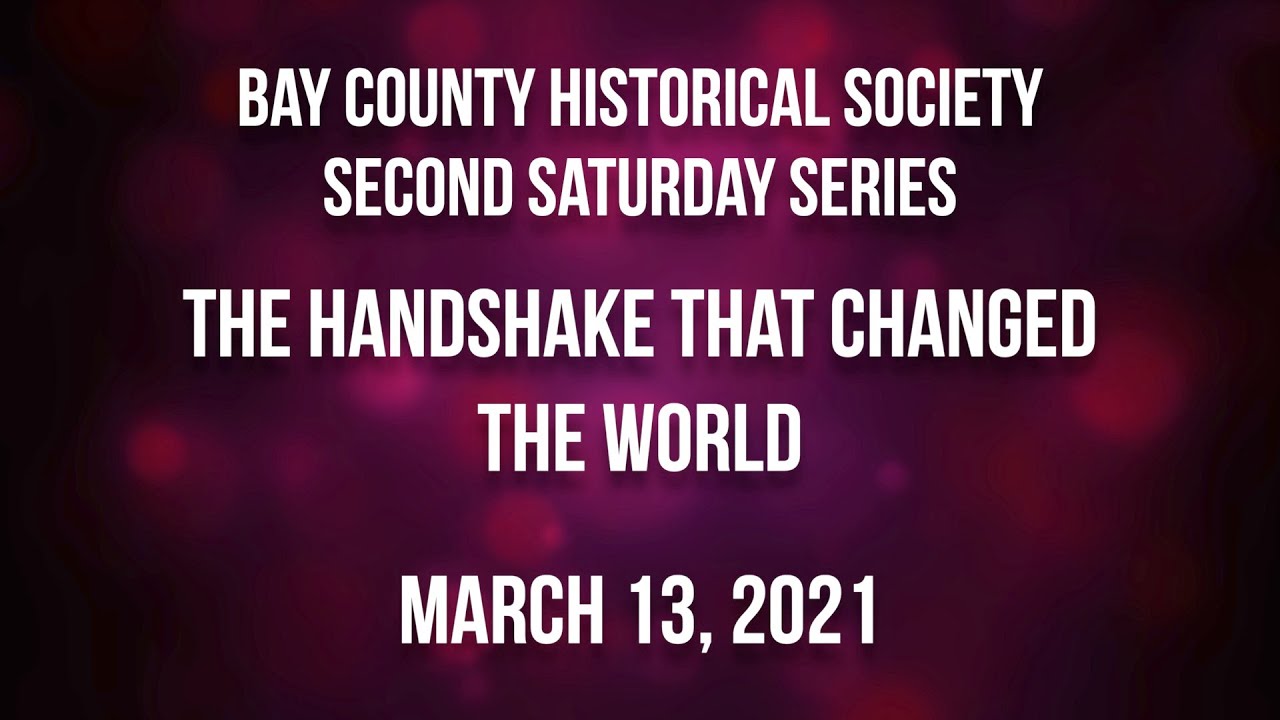This image is an advertisement poster for the Bay County Historical Society's "Second Saturday Series" event. The poster's text is designed in bold, uppercase white letters with a shadow effect, making it prominent against the abstract background. The text is spaced across five lines, reading: "Bay County Historical Society," "Second Saturday Series," "The Handshake That Changed," and "The World," with the date, "March 13th, 2021," at the bottom. The background is a gradient mix of colors, predominantly shifting from black at the corners and edges to shades of magenta, dark orange, and purple toward the center. Blurry, circular shapes in various shades of red and magenta add to the abstract, out-of-focus appearance, and contribute to the overall dreamy and artistic aesthetic of the poster.